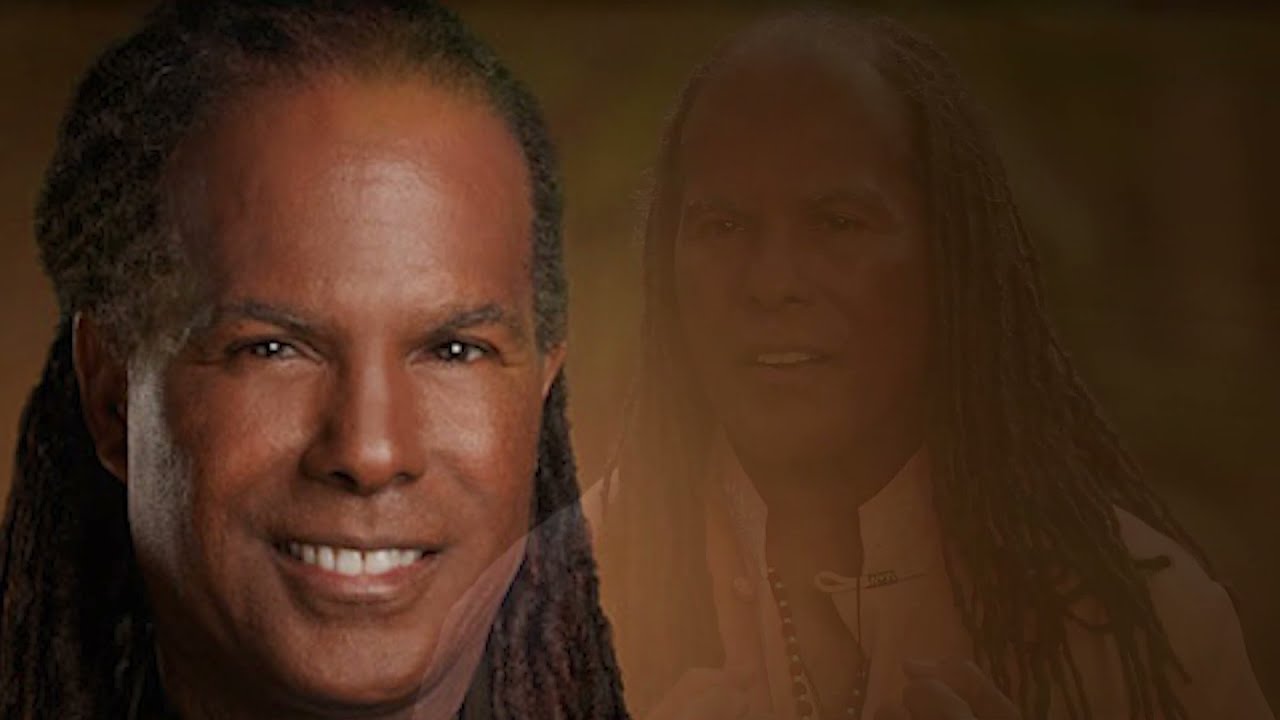The image depicts a close-up of a man with dark skin and long, braided curly hair extending to his chest, adorned with hints of gray and lighter brown tones. Positioned on the left, he smiles gently, revealing his top teeth, while sporting a white shirt with a tall collar, partially unbuttoned to show part of his chest. His hands are raised to his necklace area, fists clenched. On the right, a more translucent version of himself appears, seen from a slightly different angle, as though fading into the background, reinforcing the dual view of the same man.